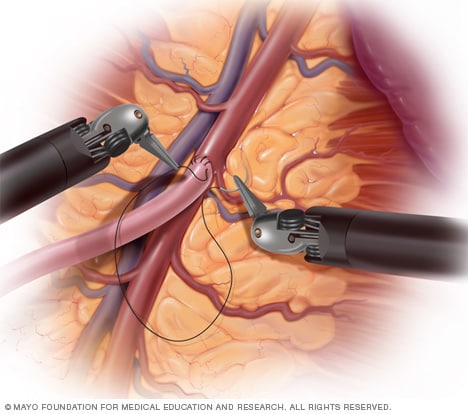This detailed medical diagram, sourced from the Mayo Foundation for Medical Education and Research, depicts a complex vascular surgery. The image portrays the interior of a human body, highlighting two prominent veins – the vein on the right is red, while the left one is blue, running diagonally from the bottom left to the top right of the frame. Surrounding these veins are light-colored swirls and muscle lines, set against a background of yellow tissue. Central to the illustration are two black surgical tools with silver tips, emerging from opposite sides. These tools are engaged in the delicate task of sewing a red tube, likely a blood valve or vein, onto another red tube with precise black stitches, showcasing the intricate method of vascular repair.